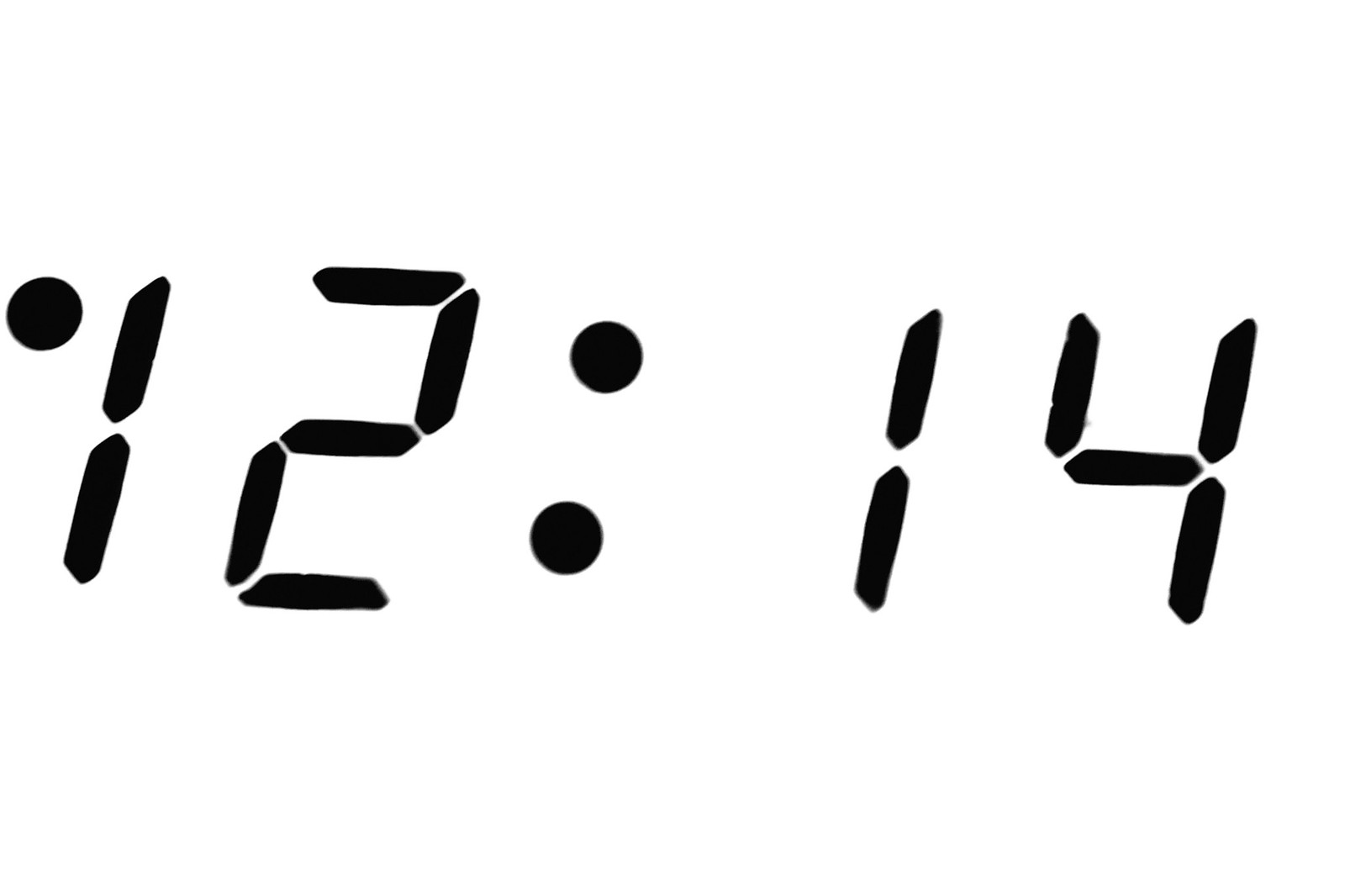This image features a set of black digital-style numbers appearing on a stark white background, resembling the display of an LED clock. The numerals "12" and "14" are prominently displayed, slightly leaning to the right in a canted manner. Positioned to the left of the digit '1' in "12" is a single black dot. Centrally located between the "12" and "14" are two black dots, resembling a colon that typically separates hours from minutes. The overall visual presentation suggests a minimalist and precise digital time display, reading "12:14," though no additional context or text is provided.